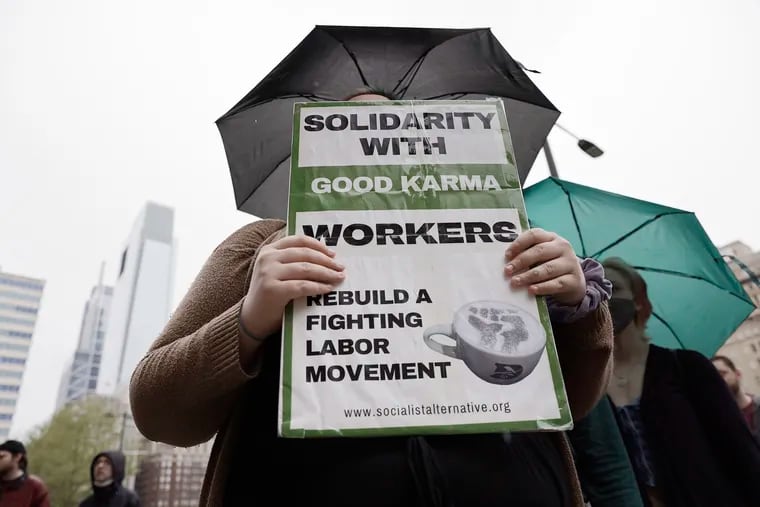This wide rectangular image captures the intensity of a protest from a below angle, showcasing the central focus on a person holding a tall rectangular sign. The protestor, clad in a long-sleeved brown sweater, firmly grips the sign with fingers horizontally overlapping its edges. Above them, a black umbrella shields against the elements, while the bright green sign vividly stands out. The sign's top section features a white rectangle with bold black lettering stating "Solidarity With," followed by "Good Karma" in prominent white letters. Further down, another white square bears the message "Workers Rebuild a Fighting Labor Movement" in black lettering, accompanied by the image of a mug with a distinct emblem. Below this, the sign displays the URL "www.socialistalternative.org."

The outdoor scene is characterized by a white sky and glimpses of buildings or skyscrapers peeking from the bottom left-hand corner, along with the green foliage of a tree. Two bystanders, one in a black hood, add to the bustling atmosphere. The wider crowd support at this apparent protest includes a visible person holding an umbrella, reinforcing the collective solidarity depicted.